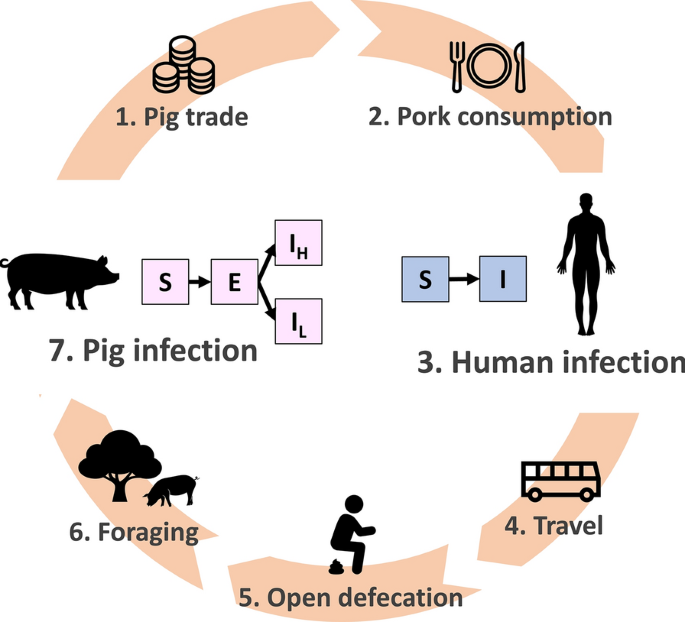The image is a detailed, circular graphic that illustrates a seven-step process numbered from 1 to 7. Starting at the top left, it begins with:

1. **Pig Trade**: This section includes an artwork depicting stacked coins, symbolizing trade or commerce involving pigs.

2. **Pork Consumption**: To the right, this part features a visual of a plate, fork, and knife, indicating the consumption of pork by humans.

3. **Human Infection**: Below, there is an artwork showing a person in black, accompanied by the letters 'S' and 'I' connected by an arrow, suggesting the transfer of infection from pigs to humans.

4. **Travel**: Further down, there's an image of a bus, representing the spread of infection through human movement.

5. **Open Defecation**: To the left, an illustration shows a person squatting with excrement beneath them, highlighting the issue of open defecation.

6. **Foraging**: This segment displays a pig digging near a tree, symbolizing pigs searching for food which can be contaminated.

7. **Pig Infection**: Lastly, at the bottom left, an artwork depicts a pig with blocks that read 'S to E,' 'E to IH,' and 'E to IL,' illustrating various stages of infection within pigs.

The caption effectively combines details from both sources, creating a comprehensive and vivid description of the circular graphic.